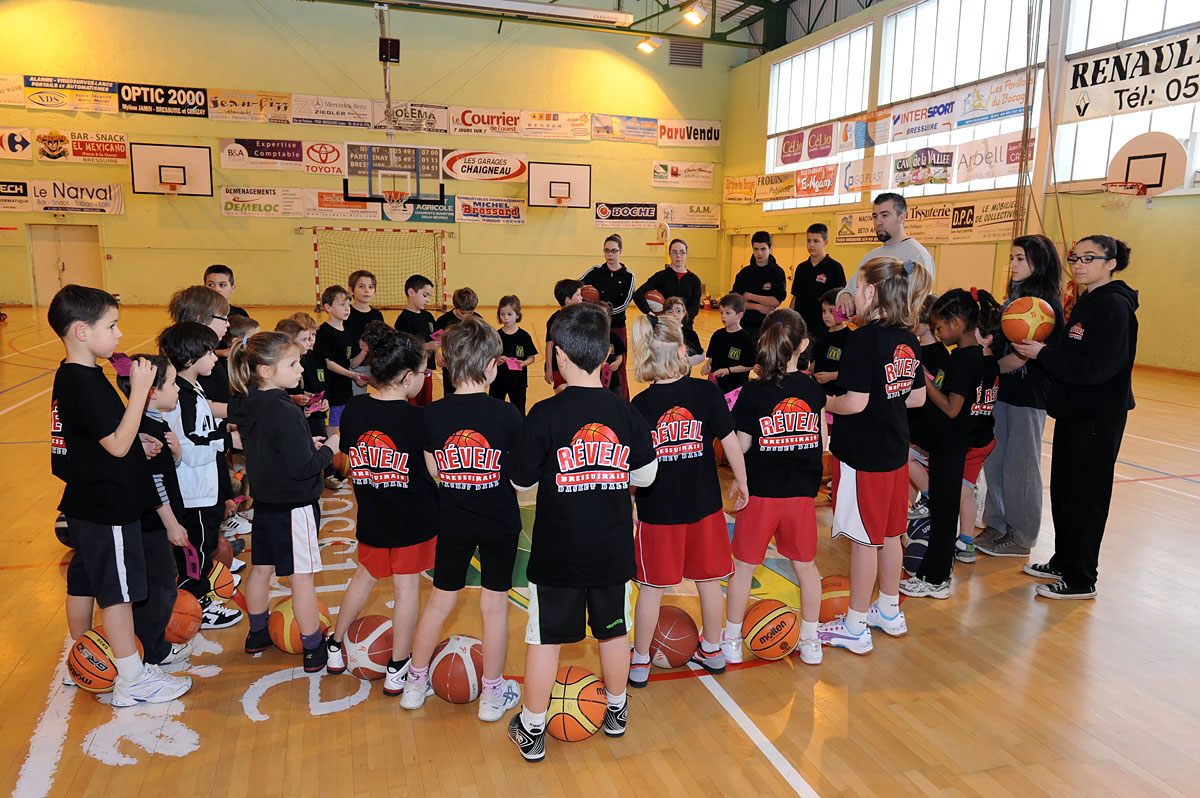In this image, a youth basketball team is gathered in a gymnasium with shiny wooden floors, light green to yellow walls, and numerous signs and banners. The group, composed of about 30 children and several adults, forms an oval-shaped circle with basketballs placed between their legs. The kids are around 8 to 10 years old, wearing black t-shirts with a basketball graphic and the word "Reveal" on the back. Some children have red and black tennis shoes, and you notice a mixture of ethnicities, including Caucasian, Black, and Asian children. On the right edge, a woman with black hair in a bun and glasses holds a basketball. In the background, you see basketball nets and large windows along the right wall, with vibrant banners promoting different businesses hanging throughout the gym.